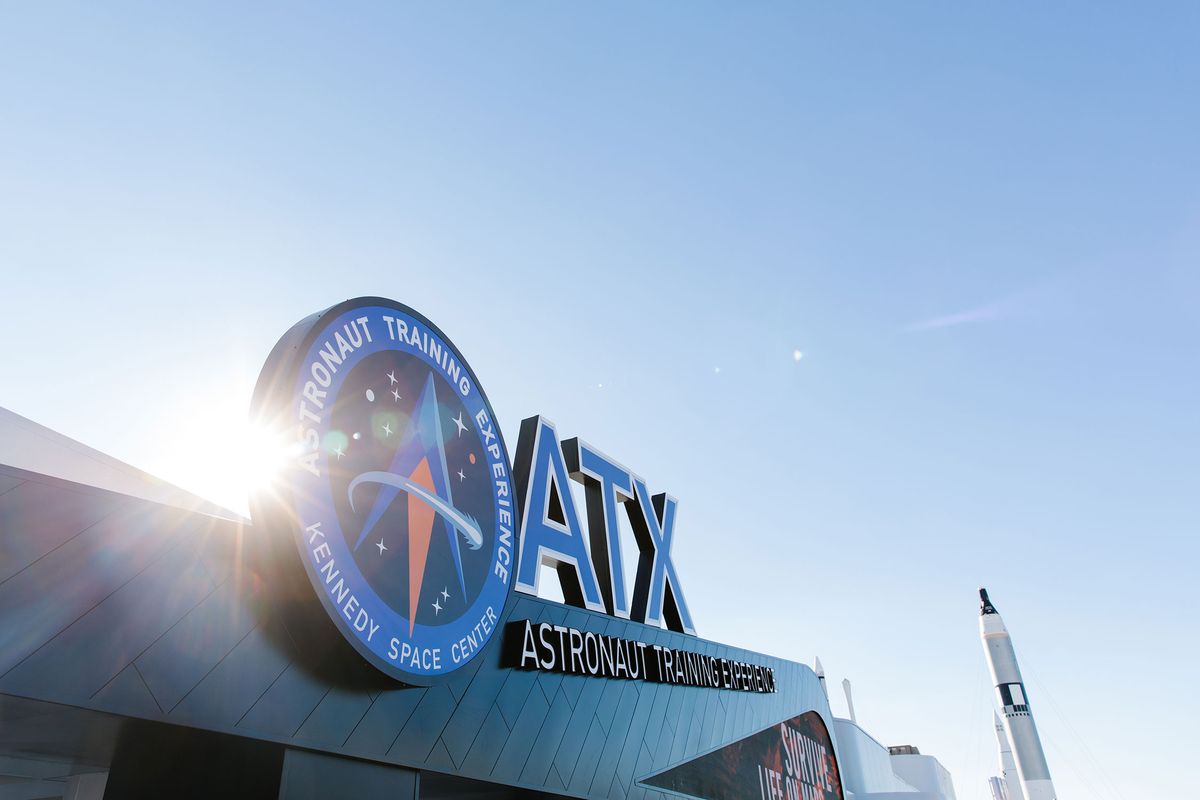In this detailed photograph, we observe the exterior façade of a building under a clear, light blue sky. Prominently displayed on the building is a large, circular sign with the blue logo, "Astronaut Training Experience Kennedy Space Center," accompanied by an icon, and to its right, large letters reading "ATX Astronaut Training Experience." Below this large header, a blue wall stretches across the building front. The bright, shining sun is positioned to the left of the circular sign, casting visible rays and enhancing the sunny, clear day ambiance. To the right of the building, a gray rocket with a black tip stands prominently in the foreground, with a smaller white rocket visible behind it. The rooftop also features an orange sign with the phrase "Survive Life on Mars." The photograph captures both the dynamic presentation of the astronaut training center’s signage and the fascinating details of the surrounding space-themed elements.